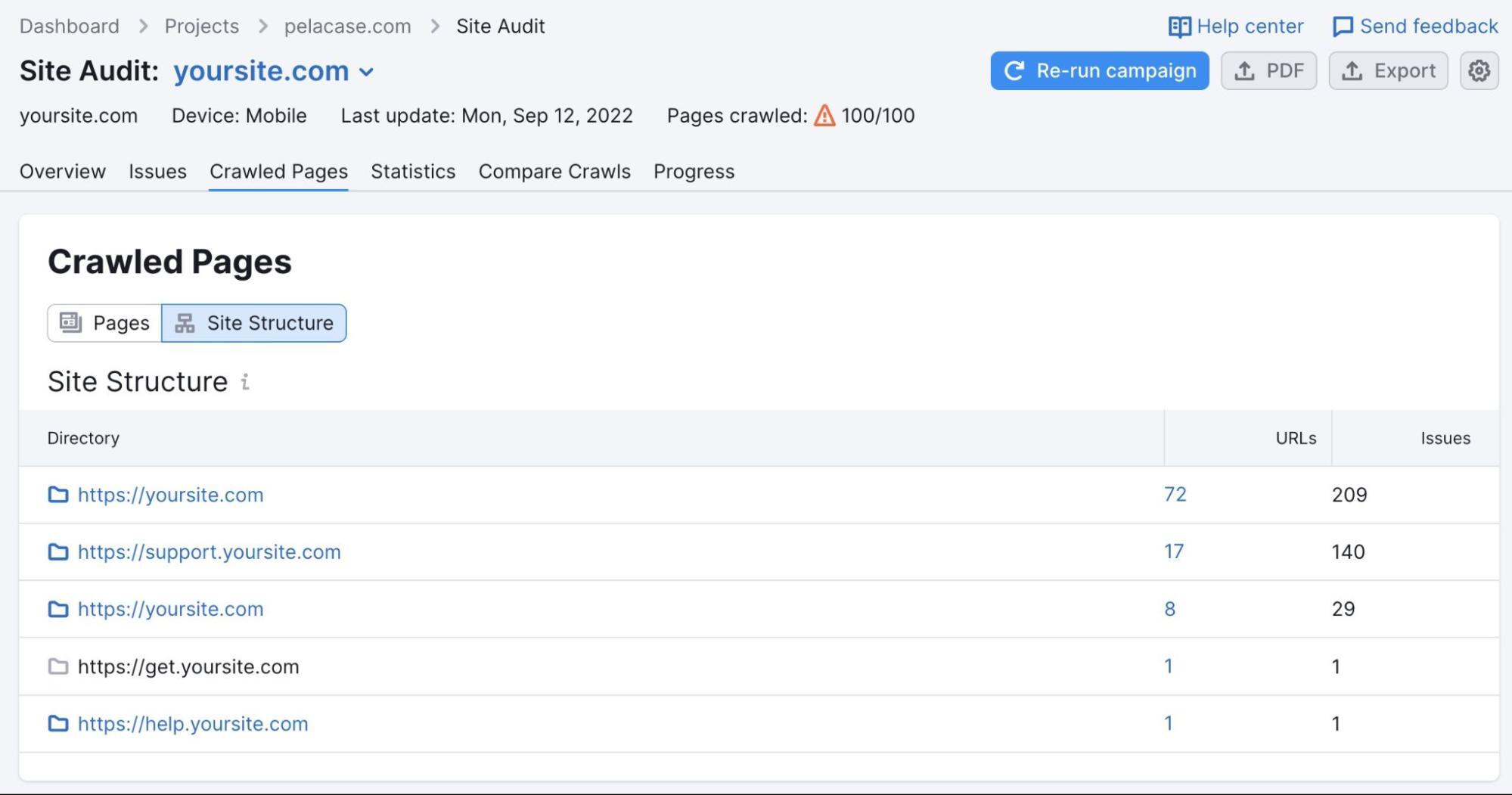The image displays a dashboard interface on a light gray background. At the top, the header reads "Dashboard - Projects - Pellicase.com - Site Audit." Below that, it mentions "Site Audit - callingyour.site.com." The site being audited, "your.site.com," is listed with the last update date specified as Monday, September 12, 2022. It also states that 100 out of 100 pages have been crawled.

The main sections includes tabs labeled "Overview," "Issues," "Crawled Pages," "Statistics," "Compare Crawls," and "Progress." At the top right corner, there are options for "Help Center," "Send Feedback," "Rerun Campaign," "PDF and Export," and a settings button.

Below these sections, a white box titled "Crawled Pages" contains buttons: a white button labeled "Pages" and a blue button labeled "Site Structure." Underneath, another section labeled "Site Structure" within a light gray box presents three columns: "Directory," "URLs," and "Issues."

From left to right, the columns lists:

- "your.site.com" with 72 URLs and 209 issues.
- "support.your.site.com" with 17 URLs and 140 issues.
- "your.site.com" with 8 URLs and 29 issues.

The detailed layout and information provided suggest a comprehensive audit of the website’s structure and issues.